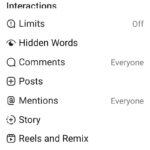The image is a blurry screenshot of the "Settings" section in the Instagram app. At the top of the screen, there is a title labeled "Interactions" on the left. Below this title, a series of categories are listed:

1. **Limits**: Displayed on the right as "Off."
2. **Hidden Words**: Accompanied by an eyeball icon on the left.
3. **Comments**: With a text bubble icon, and the setting on the right indicated as "Everyone."
4. **Posts**
5. **Mentions**: Identified with an "@" symbol, with the setting on the right shown as "Everyone."
6. **Story**: Shown with a dotted circle and a plus sign icon.
7. **Reels and Remix**

Each category is paired with a relevant icon that represents its function, making it easier for users to understand the settings related to interactions on their Instagram account.